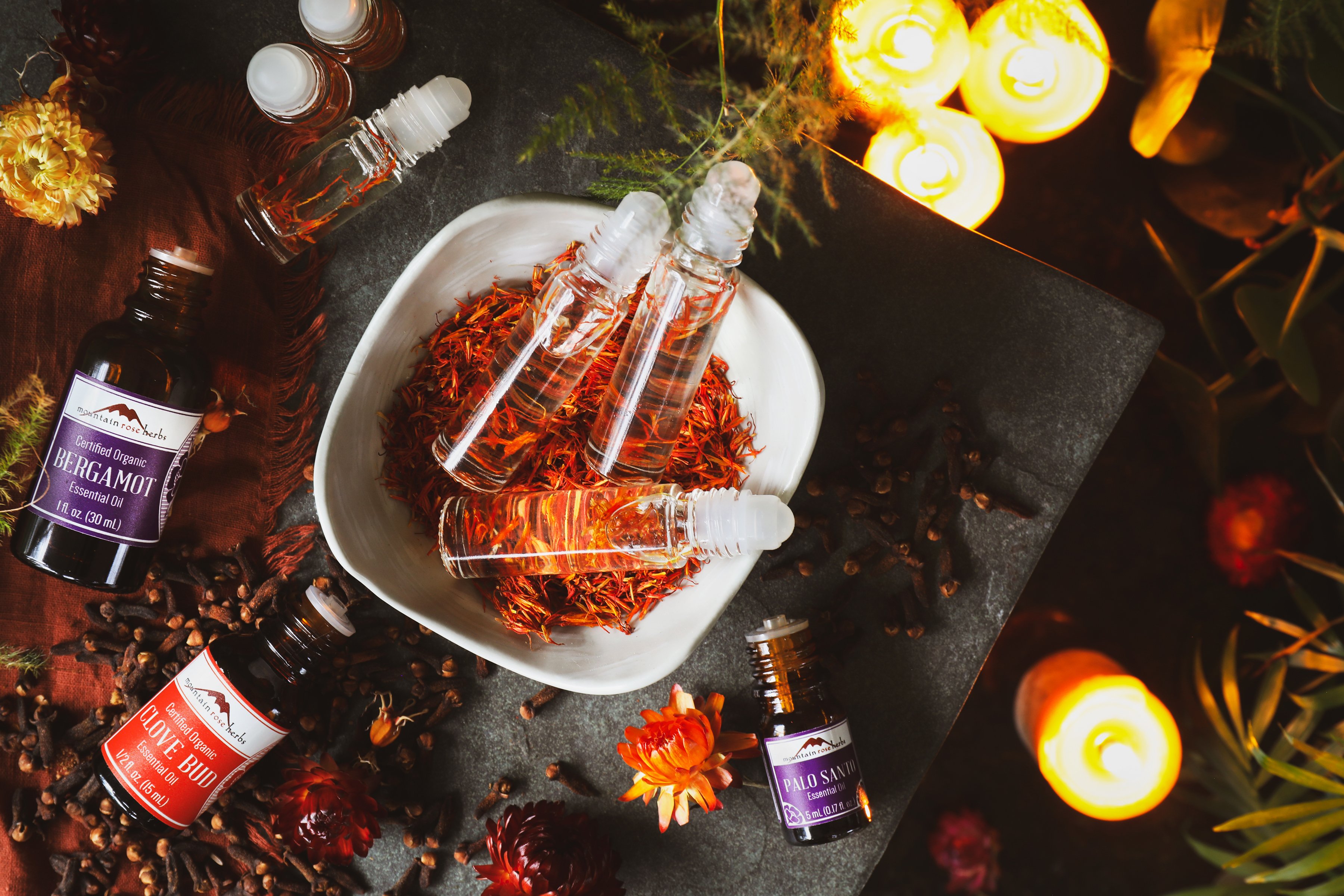The photograph captures an overhead view of an aromatic display centered on a white bowl filled with vibrant orange flower petals, resembling potpourri. Nestled within the petals are several transparent glass perfume bottles, each topped with a white transparent lid. Surrounding the bowl, there are darker bottles, some adorned with purple labels indicating Bergamot essential oil, and others with red labels, such as Clove Bud. Also noticeable is a bottle labeled Palo Santo with a purple label. Lit scented candles are positioned to the right side of the image, enhancing the soothing ambiance. The bowl rests on a rectangular gray stone and cloves are scattered across the table, adding to the perfumery and skincare-themed setting, which exudes a festive, fragrant essence.